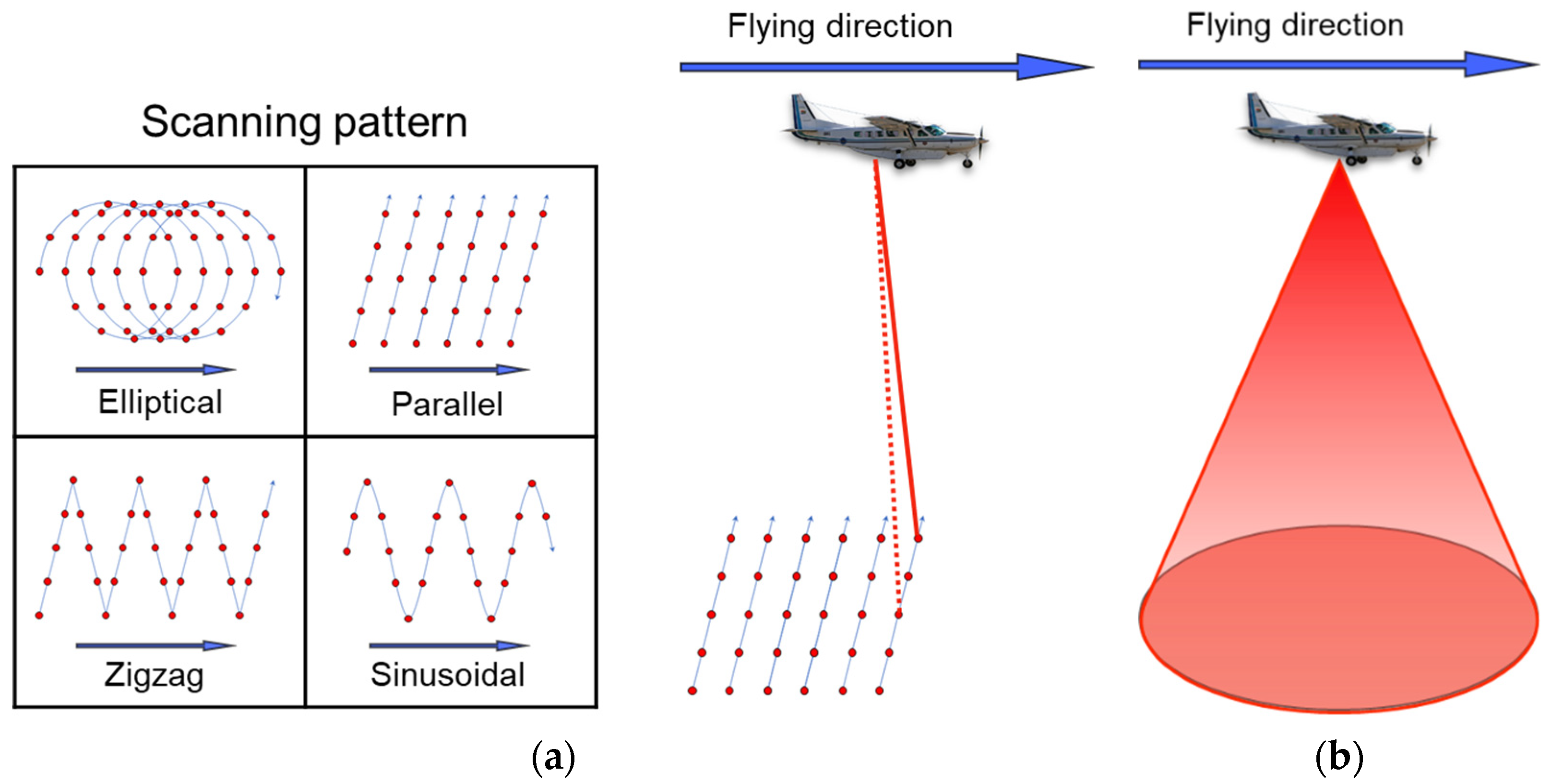The image is a detailed scientific chart demonstrating different scanning patterns and directional behaviors of aircraft technology. On the left, there is a four-panel block labeled "scanning pattern." Each panel within this block depicts a different scanning method: elliptical, characterized by spiral rings with red dots; parallel, with six diagonal lines also marked with red dots; zigzag, featuring repetitive up-and-down straight lines with red dots; and sinusoidal, showing loosely formed, undulating lines with red dots.

In the middle of the image, the term "flying direction" is featured prominently, pointing to the right. Below this text, there is a depiction of two airplanes flying towards the right, emphasized by a blue arrow labeled "flying direction." The first airplane has a solid red line and a dotted red line extending downward to a grid field, which comprises parallel lines, similar to those in the four-panel block. The second airplane is shown casting a widening red cone over the area below, suggesting a scanning action. The imagery collectively illustrates the aircraft scanning patterns and their application in monitoring ground areas.